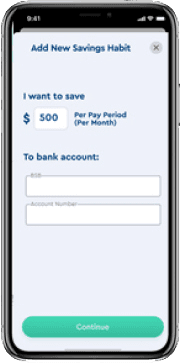A screenshot captured on a smartphone displaying a financial application interface. The phone is encased in a black protective cover, with discernible edges framing the screen. A black bar runs along the top, featuring indicators for time, Wi-Fi, and battery status. The image is notably blurry and out-of-focus, reducing legibility.

Central to the screenshot is a pop-up overlay titled "Add Savings Habit," highlighted in blue with an 'X' for closing the window in the corner. The interface suggests a financial goal, stating "I want to save" followed by a dollar sign and a text box containing the number 500. This goal is defined on a per pay period or per month basis to be deposited into a bank account. Below these details are two empty white boxes bordered in gray. A prominent round, turquoise 'Continue' button is positioned at the bottom.

The overall low-quality and blurred nature of the image suggests it could be an advertisement mock-up, possibly for web or print media, or a screenshot from a how-to video demonstrating the app's features.